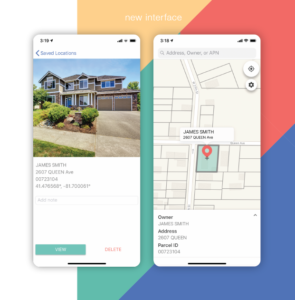This screenshot is from a website offering directions. The layout features a vertical rectangular background. At the top left, there's an orange triangle pointing to the top left, with the text "New Interface" in white. Below that, there's a color-gradient rectangle, transitioning from red at the top right to blue-green at the bottom left, and ending with a dark blue triangle at the bottom corner.

In the foreground on the left side, there's an image of a large tan house with a two-car garage. The address displayed is "James Smith, 2607 Queen Ave." Below the address, the text is too small to read. At the bottom of this section, there are two options: "View" on the left (highlighted) and "Delete" on the right.

Adjacent to this, there is a vertical rectangle featuring a picture of a map. The map has a blue rectangle highlighted and a red dot pin indicating the specific location of the address.